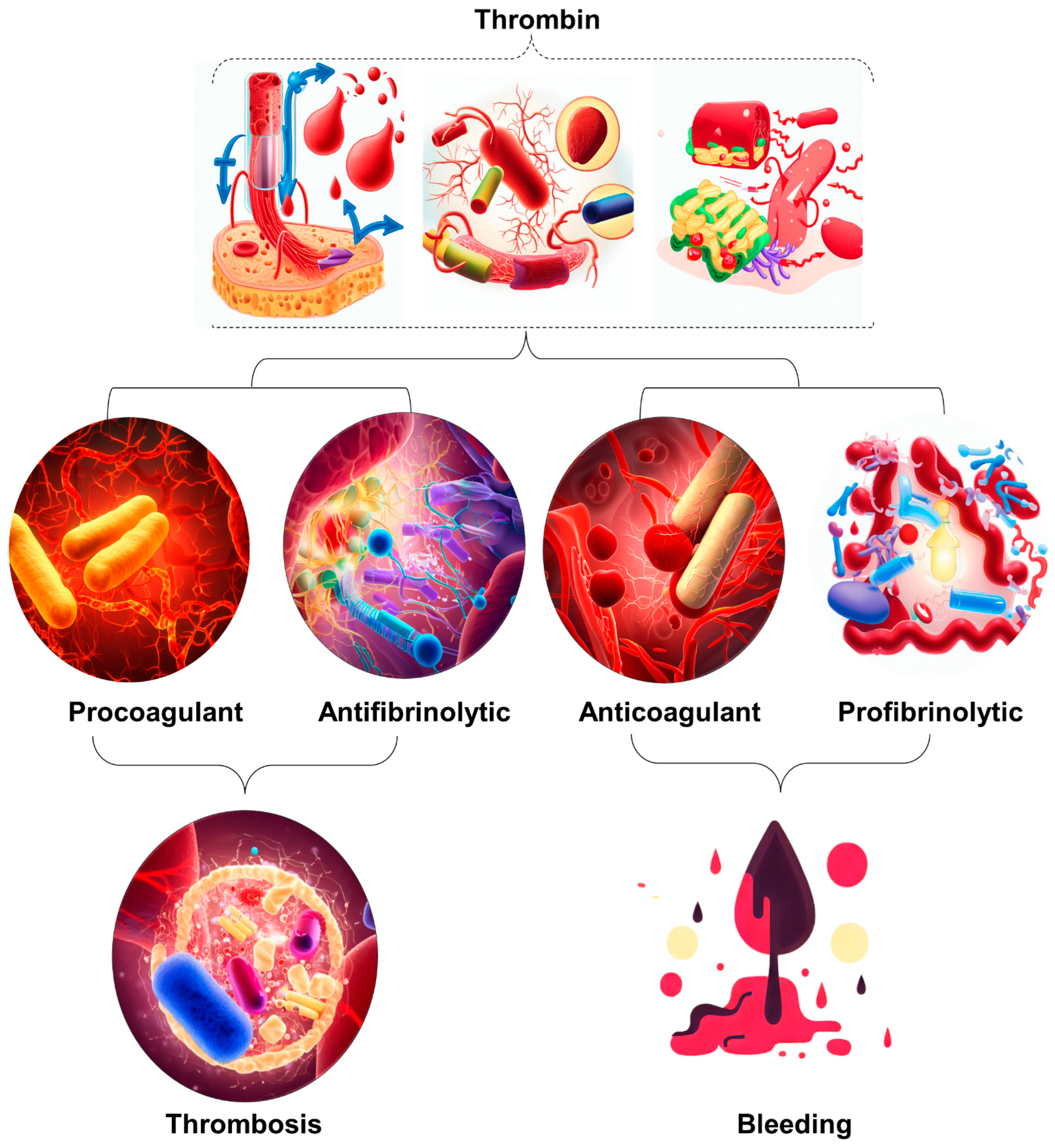The image illustrates various processes within the human body related to blood, using detailed and colorful diagrams. At the top, "Thrombin" is prominently labeled above three illustrations depicting blood flow, represented by two blood drops and a tube, as well as blue arrows indicating the direction of flow. Below, a complex diagram showcases blood vessels and tubes, followed by another with additional tubes and a cylinder. 

In the middle row, four diagrams are presented side by side. The first, labeled "Pro-Coagulant," features a circular image with three yellow tube-like structures resembling sausages, surrounded by numerous lines. Next, a diagram under the title "Anti-Fibrinolytic" displays an assortment of blue and purple tubes. The third illustration, labeled "Anti-Coagulant," contains grayish-brown tubes and what appear to be red blood cells. Lastly, the "Pro-Fibrinolytic" diagram showcases squiggly tubes and orbs.

At the bottom, two additional diagrams are shown. The "Thrombosis" image is a circular diagram containing a smaller circle filled with various tubes and colors. Next to it, a "Bleeding" illustration features a teardrop-shaped blood drop in purple and pink hues, surrounded by smaller circles in purple, pink, and white. The overall depiction aims to convey the complexity of blood-related processes within the human body.